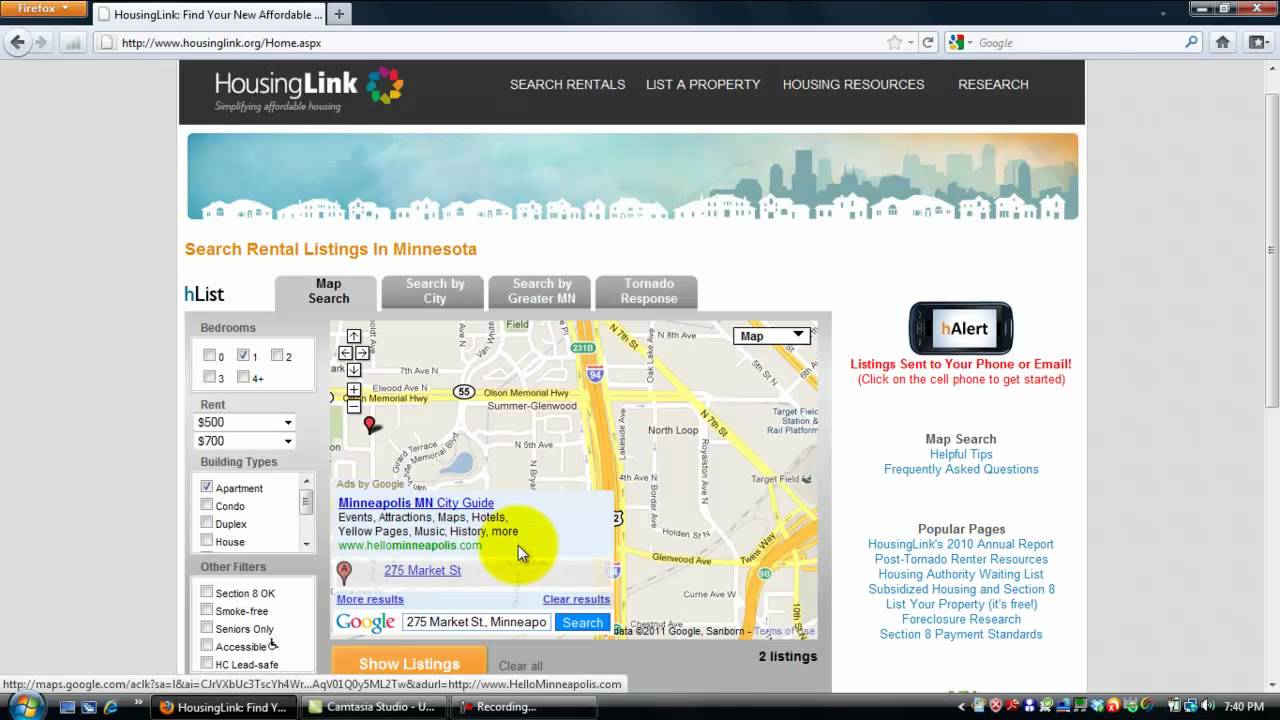This detailed caption beautifully describes the layout and elements of the webpage:

---

The image shows a webpage viewed through the Firefox browser. In the top left corner, the word "Firefox" is visible. Beside it, a tab labeled "Housing Link: Find Your New Affordable..." is open. Moving right, the top right corner features three control buttons: minimize, fullscreen, and close (X). Below these, on the left side of the interface, are backward and forward navigation arrows, followed by a search bar. The search bar contains the URL "http://www.housinglink.org/house.aspx". To the right of the search bar, there is a bookmark icon and a refresh button.

Within the main body of the webpage, the title "Housing Link" appears on the left side, with the tagline "Simplifying Affordable Housing" underneath. Adjacent to these, towards the right, are four navigational tabs reading: "Search Rentals," "List a Property," "Housing Resources," and "Research." Beneath these sections, there is an illustration of buildings, contributing to the aesthetic and thematic context of the page.